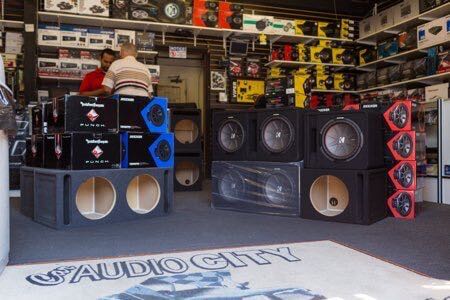This image showcases the vibrant interior of an audio store, captured from an angled perspective. In the center foreground, a large white mat emboldened with "Car Audio City" anchors the scene, laying atop grey carpet. To the left, stacked black and blue speaker boxes dominate, while black speakers, including one wrapped in plastic, are prominently displayed to the right. The speaker boxes have distinct black and blue designs, alongside gray boxes revealing a hollow wood interior, presumably containing plywood. 

Further, a black display case houses more boxed speakers, and larger exposed speakers with neodymium centers are positioned conspicuously, accompanied by informative red signs detailing their drivers. Shelves crammed from floor to ceiling with varied stock—including white, black, and yellow boxes—wrap around the store, showcasing a broad range of stereo equipment.

The bustle in the store is heightened by two customers near the back, possibly at a counter. One wears a striped brown and tan shirt with his back to the camera, while the other, facing us, sports a bright red shirt and dark hair. A man in a white polo shirt with thinning hair appears to be receiving assistance from another employee. The scene is a detailed snapshot of the lively and well-stocked interior of Car Audio City, capturing the essence of its packed shelves and diverse audio offerings.